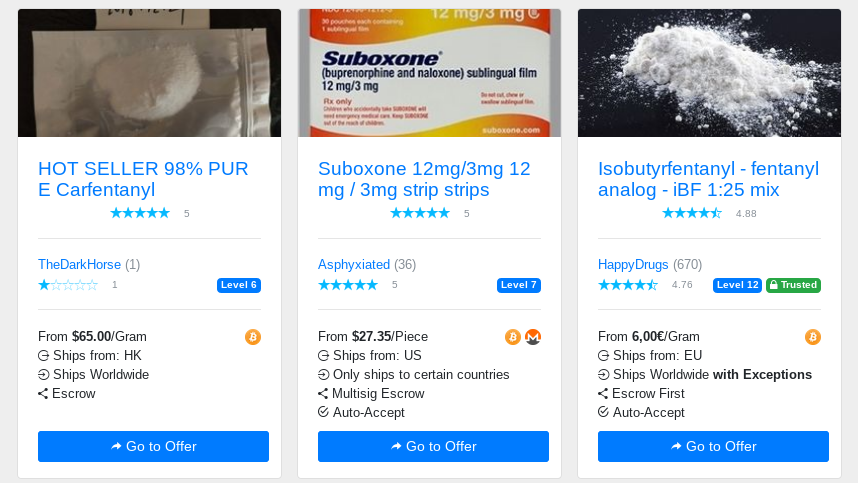**Detailed Caption:**

The image showcases three different offer listings, each meticulously organized with various details.

1. The first listing to the left features "Hutz Cellar" in prominent blue capital letters. Beneath it, "98% PUR" is indicated, followed by the letter "E." Below this, "Carr Fentanyl" is presented in standard, grammatically correct lettering. The product rating is clearly visible with five blue stars accompanied by a gray number "5." All these elements are enclosed within a light gray border. Beneath this text block, there is the name "The Dark Horse" written in blue, with a light gray number "(1)" next to it. Below, five outlined stars are displayed, with the first star filled in blue, indicating a one-star rating by the seller. To the right of this is a dark blue rectangle with rounded corners, containing white text that reads "level 6." Further down, a light gray divider separates the next section, which states "from" in black writing, followed by a bold price of "65.00/gram." Below this information, it specifies "ships from: HK" and "ships worldwide." At the bottom of this listing, "escrow" is noted, followed by a long blue rectangle featuring white text that says "go to offer," accompanied by a right-pointing arrow on the left side.

2. The second listing advertises "Suboxone" in blue text. It details the product as "Suboxone 12MG/3MG12MG/3MG strip" followed by the word "strips." This listing boasts a perfect rating with five filled blue stars and a light gray number "5." A light gray line divides this section from the following. Below, another five-star rating is displayed with the number "36" in light gray parentheses, indicating the number of reviews. Like the previous listing, a blue rectangular icon at the bottom with white text reads "go to offer," alongside a curved arrow.

The structure and colors of the elements, such as stars, borders, and dividers, effectively organize the information and enhance readability, ensuring each listing is comprehensively detailed.